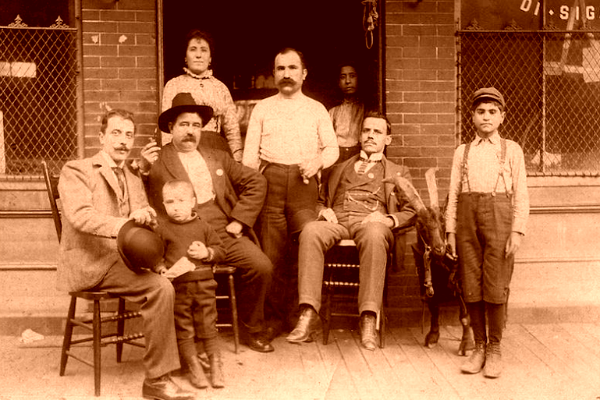This vintage sepia-toned photograph captures a late 19th or early 20th-century scene, likely in front of a small business establishment. The image features eight individuals posed on a wooden platform or boardwalk, set against the backdrop of a brick building with metal window grates. The group consists of six men, one young boy, and a small child approximate to three or four years old. 

On the far left, a man wearing a bowler hat, propped on his knee, sits with a young child standing in front of him. Next to him, an older gentleman donning a cowboy hat and a black suit, sits with his hand resting on his thigh. Behind this man, a woman in a high-collared dress stands. At the center of the photograph, a man stands with a prominent mustache, dressed in light-colored shirt and tan pants. Behind him is a woman who appears to be of Native American heritage, possibly a maid or servant. 

To the right, another man leans confidently back in his chair, balancing on its rear legs, dressed in an expensive suit with slicked-back hair. Standing next to him, a boy around ten or twelve years old, wears a cap, large suspenders, short pant overalls or breeches, and tall boots. A dark-colored goat with large horns stands beside this boy, adding a rustic element to the scene.

Together, they stand in front of a storefront characterized by its open doorway framed with brick columns and windows secured by steel diamond-shaped protective grids. The overall ambiance, attire, and architectural details suggest the photograph was taken around the turn of the century, giving it a distinctly historical essence.